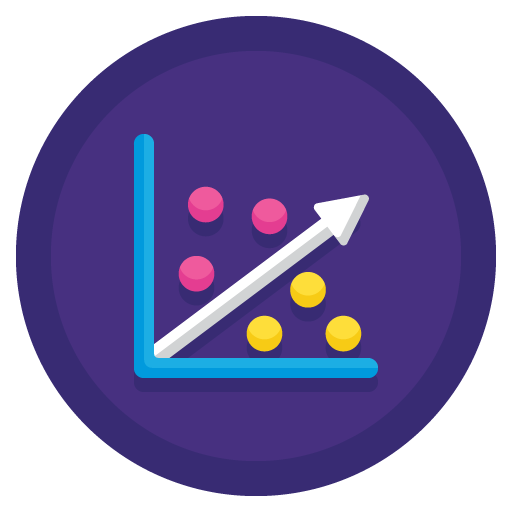This icon features a purple circular design with a darker purple border encircling a slightly lighter purple inner circle. At the center of the circle is a white XY graph, focusing on the positive X and positive Y quadrants. A linear arrow stretches diagonally along the line Y = X. Above this white arrow, there are three red spheres with a 3D texture, showcasing darker pink shading at the bottom and lighter pink at the top, creating a sense of depth. Below the arrow, three yellow spheres exhibit a similar shading effect, with darker yellow at the bottom and lighter highlights at the top. The white arrow itself has a gradient, appearing lighter on the upper left side and transitioning to a grayer hue at the bottom edge. All elements of the icon display consistent shading to enhance the three-dimensional appearance.